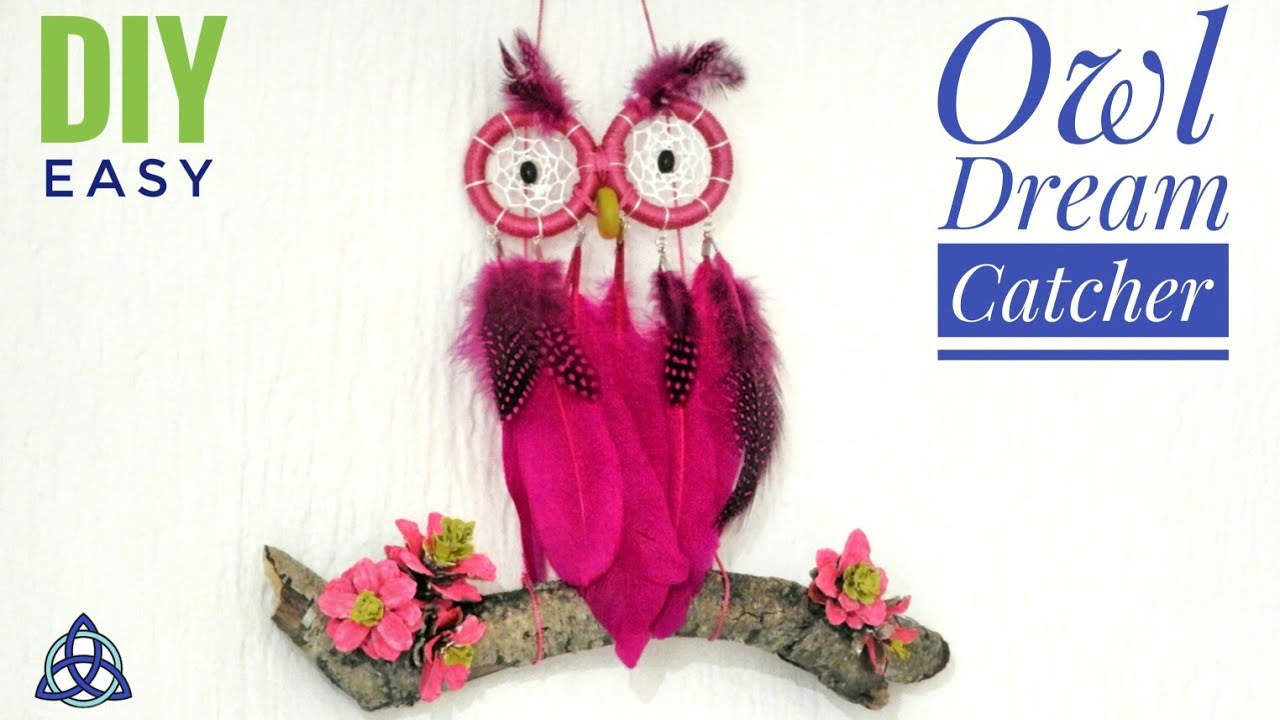This image features an intricate DIY craft project against a white background. In the upper left-hand corner, the text "DIY" is displayed in green, with "easy" written in blue beneath it. On the top right-hand corner, the words "Owl Dream Catcher" are arranged, with "Owl" in purple and "Dream Catcher" in white within a purple rectangle. In the lower left-hand corner, there's a symbol of a blue ring with three purple almond shapes superimposed onto it.

At the center of the image is a creative representation of a dream catcher designed to resemble an owl, reflecting Indigenous and Native American cultural beliefs about dream catchers as spiritual objects. The owl figure is crafted using pink feathers for its body, with small nets featuring black eyes and pink-rimmed feather eyebrows. The owl's wings are made of black feathers adorned with pink polka dots. It is perched on a brown branch which is accented by pink and yellow flowers on each side. The owl also has a small, yellow beak. 

This detailed and visually rich composition presents both the symbolic spiritual significance of the dream catcher and the creativity involved in its DIY crafting.